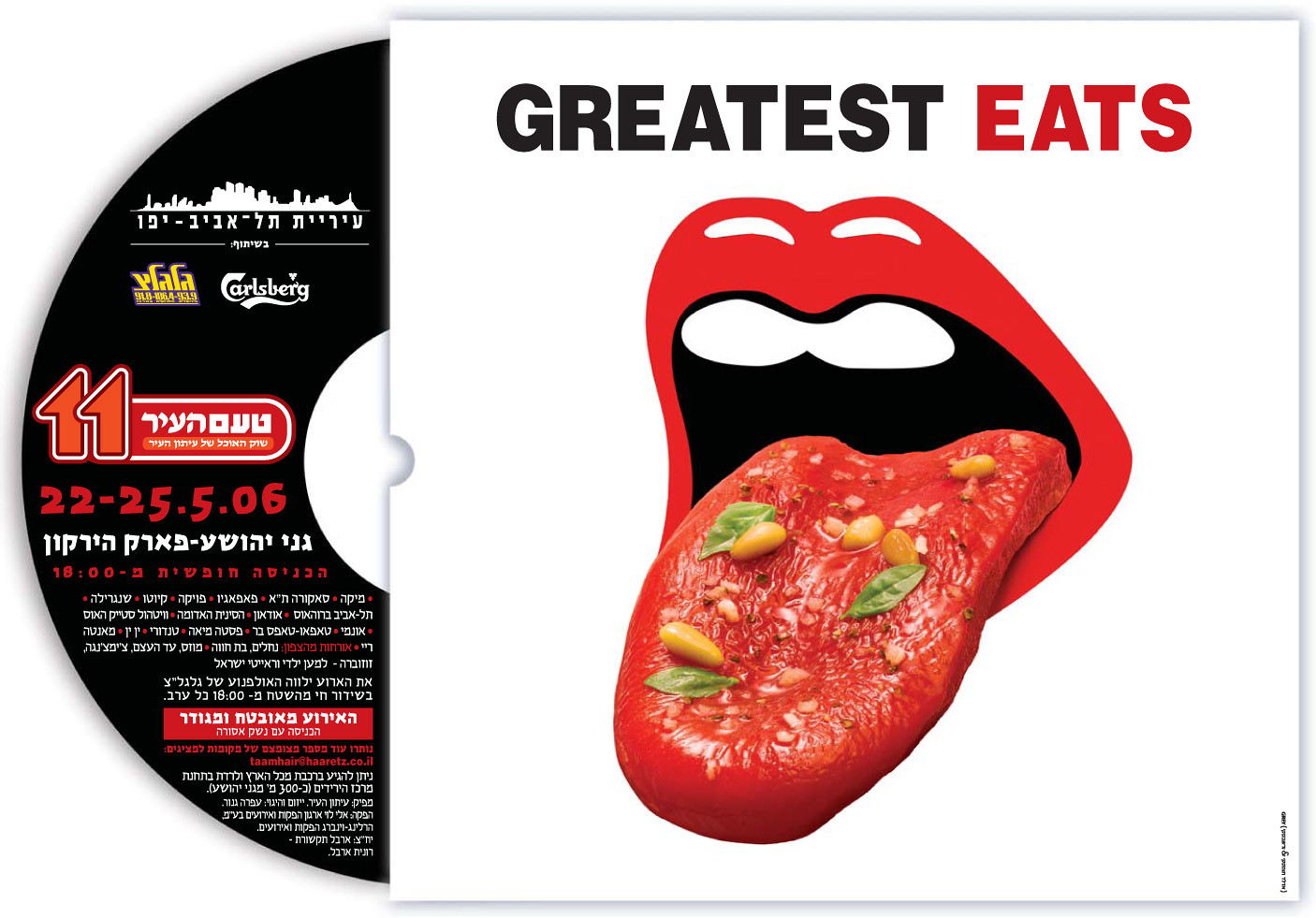The image is an album cover featuring a white rectangular sleeve with a black stylized vinyl record partially protruding from the left side. Dominantly displayed across the top of the sleeve are the words "Greatest Eats" — "Greatest" in bold black text and "Eats" in bold red text. Below this title is a cartoonish illustration of a mouth with red lips, exposing white teeth, and a black inner mouth. A realistic human tongue extends outward from the mouth, covered with various seeds and leaves, resembling food or spices. The cover's bottom right corner contains legible black font text, potentially indicating album details or credits. Foreign text, primarily in Hebrew, spans multiple lines in white and red across the artwork, hinting at its non-English origins. Additionally, the date "22-25.5.06" appears to signify a specific time period, possibly for a promotional event related to food and music. The black disk, suggesting a CD or vinyl record, also includes red and white text, with some sponsors or company names, one highlighted in gold.